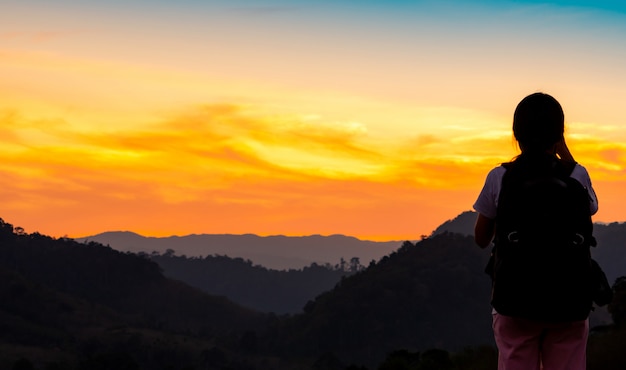The photograph captures a striking scene of a woman standing at the bottom right, seen from just above her knees up. She has her hair tied in a ponytail and is wearing a backpack, appearing in a dark silhouette. With her right hand raised, she is holding either binoculars or a camera up to her face, intently gazing at a breathtaking sunset. She is wearing red pants and seems to be walking on a trail. The sunset unfolds over multiple layers of mountains, which transition from a completely black silhouette in the foreground, to lighter shades of gray as they recede into the horizon. The sky is a tapestry of colors, starting with a bright yellow line above the furthest mountain, which gradually turns into a mix of pink and yellow. As you look higher, the sky shifts to vibrant oranges, followed by yellow, white, and finally a deep blue at the top. The scene beautifully captures the transition from day to night over a serene mountainous landscape with a valley featuring varied elevations and trees.